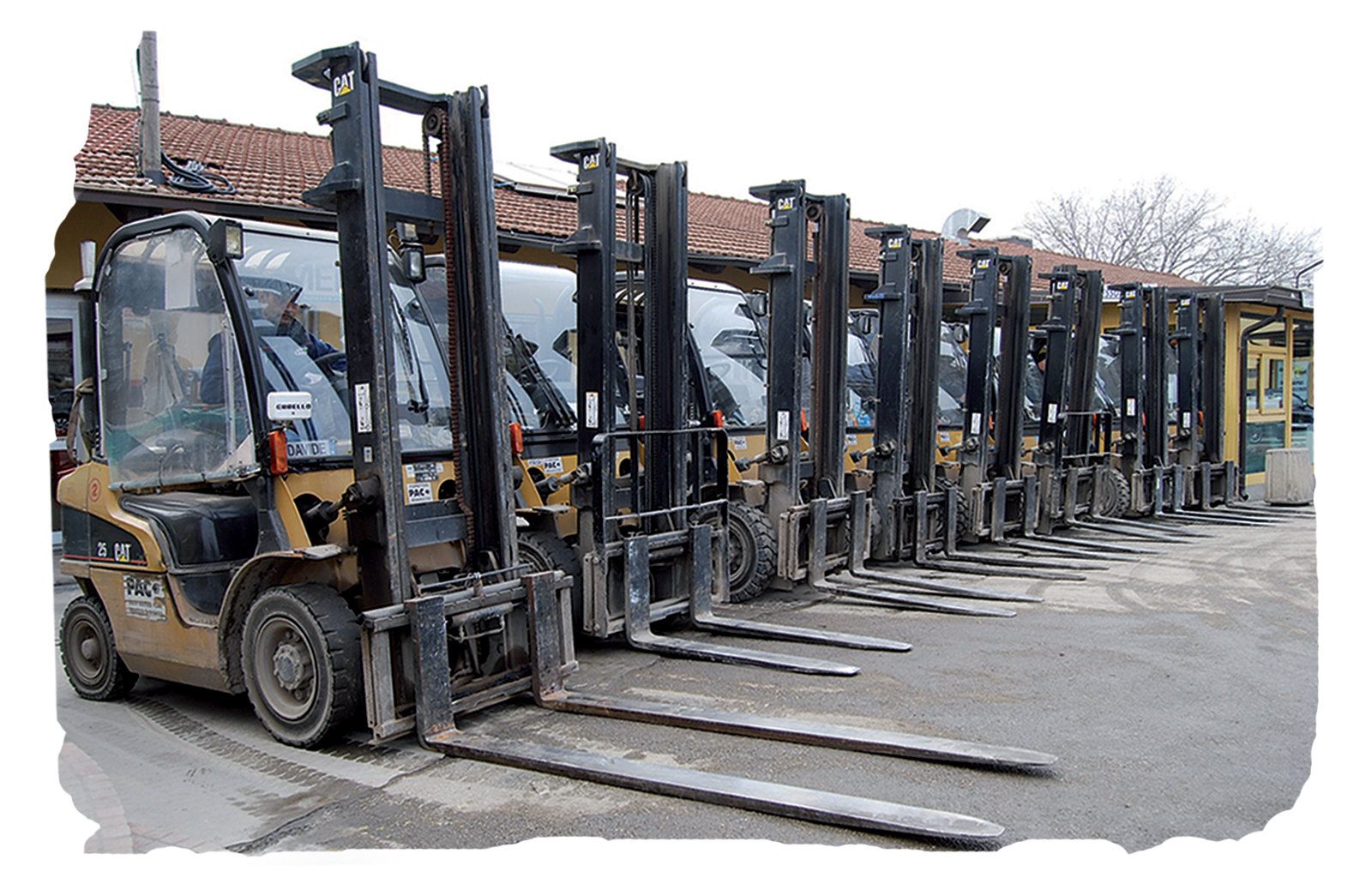This industrial photograph showcases a lineup of eight forklifts parked in a row, positioned atop a black asphalt and gray stone driveway within a concrete parking lot. Each forklift features a dull yellow base with significant machinery details: large black wheels in the front, smaller black wheels in the back, and two prominent forks extending from the front. Taller black metal frames rise from these forks, containing the chains essential for operation. Notably, the foremost forklift has exceptionally long forks, suggesting it is designed for larger loads. A man wearing a navy blue sweatshirt is seated at the controls of this leading forklift. All forklifts have yellow bodies, with canopies made of clear plastic or glass. In the background, there is a light yellow building with a brick red shingled roof, which extends as a long roof over the forklifts, ending at a small entryway booth of the same yellow color. The image portrays these forklifts as if ready for rental or use in an industrial setting, creating a sense of organized preparation.